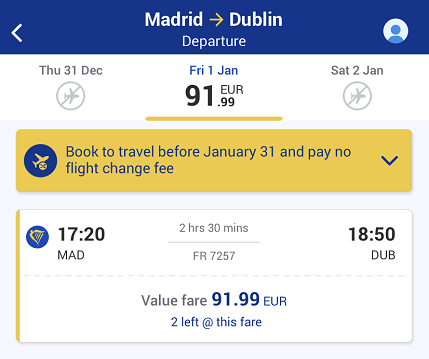This is a detailed screenshot of an online travel booking interface for a flight from Madrid to Dublin. At the top of the screen, there's a blue bar featuring the travel route: "Madrid" in white font with a yellow arrow pointing towards "Dublin," also displayed in white. Below these, the word "Departure" is written in white. On the far right of this blue banner, there is a blue profile or account icon, and on the left, there's a back arrow in white.

Immediately beneath the blue banner, the screen's background turns white, displaying three date options: Thursday, 31st of December; Friday, 1st of January; and Saturday, 2nd of January. 

For Thursday, 31st of December, and Saturday, 2nd of January, there is an icon of a small airplane encircled and crossed out, indicating no available flights on these dates. For Friday, 1st of January, there is a flight available for €91.99.

Below the date listings, a yellow drop-down banner advises: "Book to travel before January 31st and pay no flight change fee." 

Further down, a box provides specific details of the available flight: it departs Madrid (MAD) at 17:20, has a duration of 2 hours and 30 minutes, and arrives in Dublin (DUB) at 18:50. The flight number is FR7257, and the 'Value Fare' is priced at €91.99, with only two seats left at this rate.